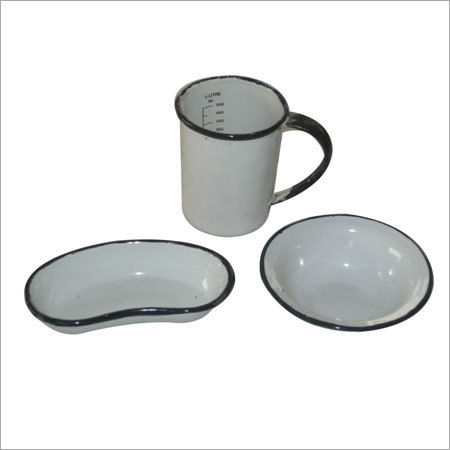The image depicts three old-fashioned white enameled dishes set against a white background. Each dish features a distinctive black rim. At the top-center of the image is a white mug adorned with measurement markings on the inside and a black handle. On the lower left is a kidney-shaped, or lima bean-shaped, disassembly bowl, similarly rimmed in black, reminiscent of a bed pan or spit cup. Positioned to the lower right is a standard, round bowl, also white with a black circular rim. All items appear to be empty, emphasizing their clean, minimalist aesthetic.